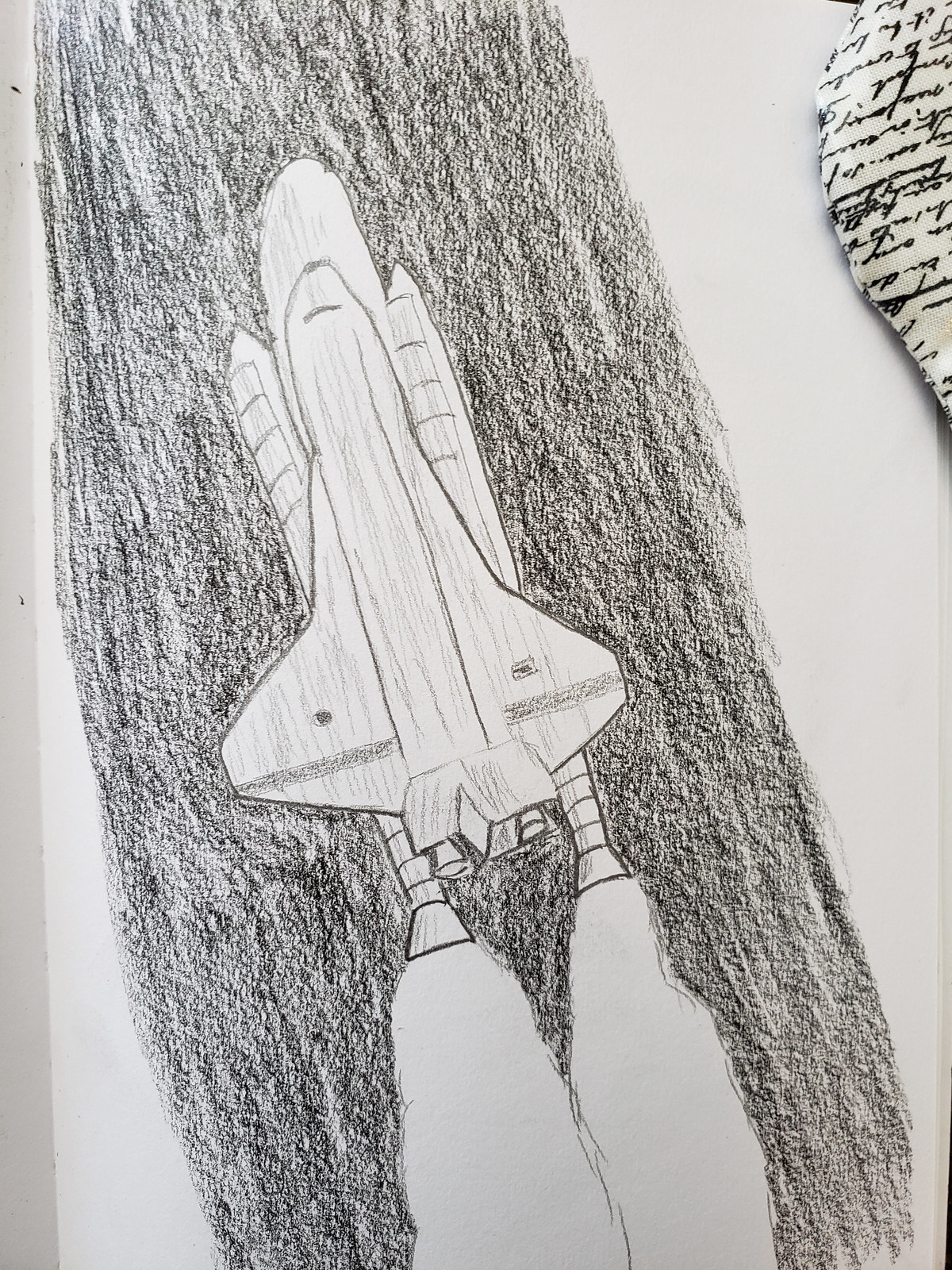This is a detailed pencil and charcoal sketch of a space shuttle blasting off. The artwork features the shuttle prominently centered, showcasing the intricate details of its structure. On each side, the two solid rocket boosters are clearly visible, with their nozzles emitting powerful flames. The main fuel tank, positioned between the boosters, supports the shuttle mounted on its back. The spacecraft is depicted in shades of gray and white, creating a stark contrast against the darker, grainy background, which suggests the vastness of space, possibly achieved through the use of charcoal or crayon. In the right edge of the composition, there is an additional element that appears to be a pad or pillow with graphic designs, subtly framed against an off-white backdrop. This juxtaposition adds a unique layer to the otherwise aerospace-focused illustration.